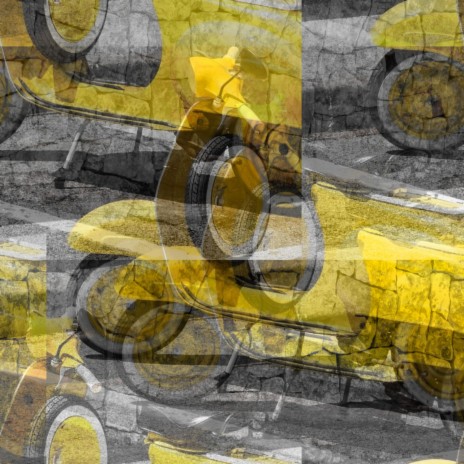The image is an abstract photographic art piece featuring multiple superimposed and fragmented views of an antique yellow vehicle, primarily in shades of yellow, black, white, and gray. The central focus is on the yellow body and white-rimmed tires with black tread. The image presents a mosaic-like break effect, making it challenging to discern specific details at first glance. Closer examination reveals the presence of a yellow fender, a whitewalled tire, and even a windshield, suggesting that the vehicle could be a motorcycle, though the sled-like undercarriage hints at an antique car. The repeated layering and mixed perspectives of the vehicle fragments blend together, creating a complex and visually intriguing abstract composition.